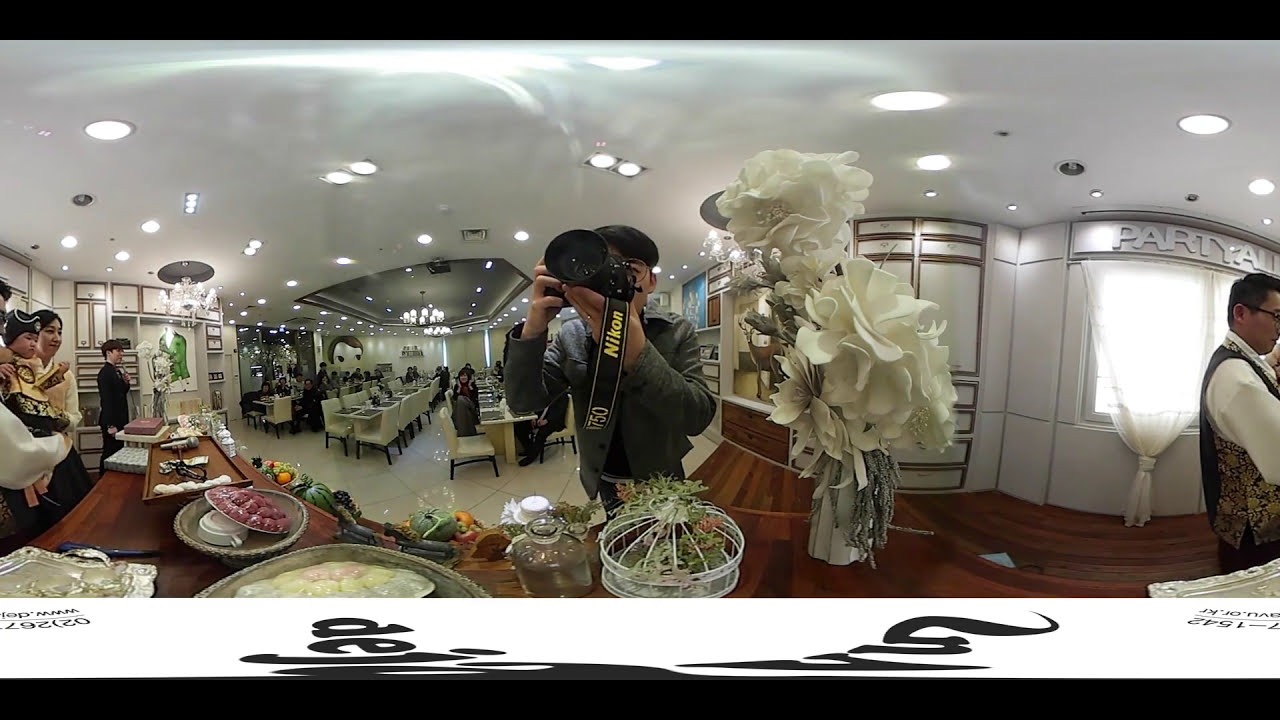The photograph captures a vibrant and detailed indoor scene dominated by white and bright elements. At the center, a man with short black hair, glasses, and a gray long-sleeve shirt is holding a large manual camera with a black and yellow strap that says "Nikon." He stands on a wooden floor, surrounded by an organized array of white tables and chairs. To his left, there is a long table lined with various platters of food, including salads and desserts, served by people behind the table. 

On the right side of the image, there is a man partially out of the frame, wearing glasses, a white shirt, and a gold and black vest. Further to the right, there is another man wearing all black and holding a microphone. The leftmost side of the image features a woman holding a baby, with another person partially obscured. 

In the background, the restaurant environment is evident with its bright, white lights hanging from the ceiling, large white life-size bouquet statues, and many white square tiles on the floor. There are multiple cabinets and spotlights illuminating the area. On the wall, there is partially visible text that includes the word "party" and an intriguing mural of a boy with brown hair. Also visible is a glass screen door. Among the tables, various people are seated, indicating a social gathering or event. The detailed interior and bustling activity suggest a lively atmosphere captured by the central figure with the camera.